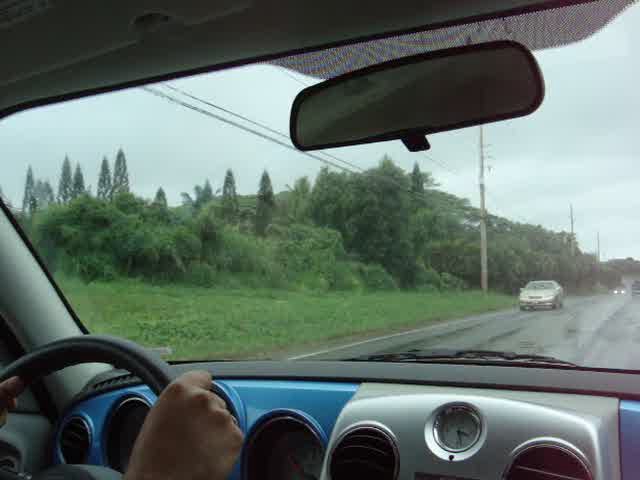A photograph taken from the inside of a car, capturing the driver's perspective as they navigate a wet road. The driver's light-skinned hands are visible on the blue and silver steering wheel, with one hand partially shown. The dashboard features a blue gauge cluster and a silver panel, with a clock situated between the central air vents. Outside, green grass lines the roadside, accompanied by pylons for electricity. To the left, dense vegetation and trees frame the scene, while another car approaches from the opposite direction on the wet road.